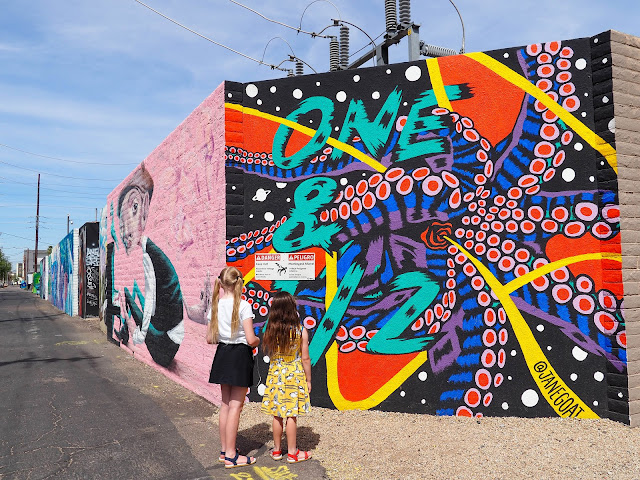The image depicts a vibrant street scene in landscape mode, featuring a contemporary photograph of a mural on the exterior wall of a potentially industrial building, devoid of windows. The focal point of the colorful mural is bold, bright blue lettering that reads "1 and 12," surrounded by an intricate design, including vivid octopus tentacles adorned with red and pink suction cups and blue and black backsides. This striking artwork is set against a wildly colorful background, featuring dots resembling planets, squiggles, circles, and patterns in red, yellow, orange, purple, and black with white polka dots.

In the foreground, two young girls, appearing to be between five and ten years old, stand in sandals and summer dresses. One girl wears a white shirt with a black skirt, while the other dons a dress with a yellow pattern. They have their backs turned to the viewer as they attentively gaze at the mural. To the left, a man is barely visible against the pink-toned extension of the mural-covered wall, which stretches further, revealing more artistic graffiti. The mural is signed with "at Jane Goat" in the bottom right corner, adding a distinct personal touch to this eye-catching urban artwork.